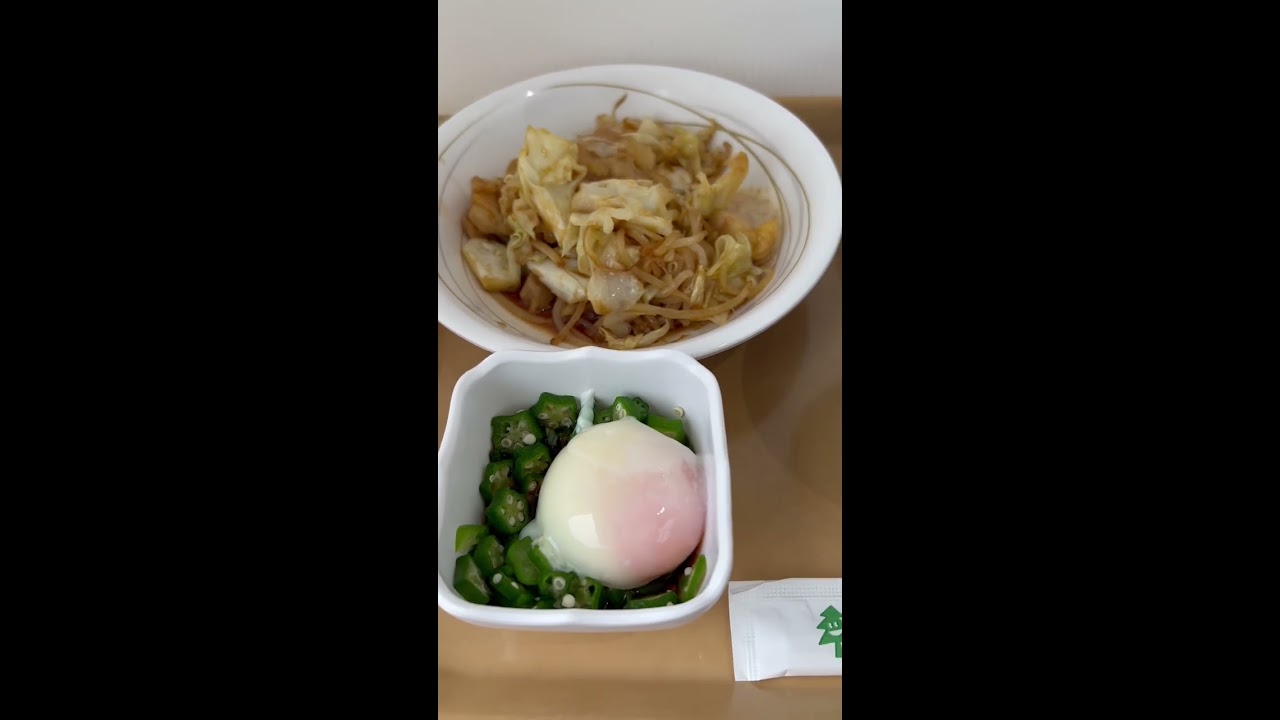The image showcases a detailed view of two bowls of food placed on a light brown wooden table, with a dark background on the left and right thirds, emphasizing the dishes. Towards the back, there is a circular porcelain bowl adorned with golden streaks, containing noodles mixed with a brown sauce, likely soy sauce or teriyaki, accompanied by scrambled eggs. In front of it is a multi-sided rectangular dish filled with chopped green vegetables, potentially okra or jalapenos, topped with a significant white item, possibly a white bun or a bulbous vegetable resembling an onion or an egg, tinged pink on the right edge. To the right of this rectangular dish sits a small white packet featuring a smiling green Christmas tree. The overall setting, which could be a preparation stage or someone's lunch, hints at an inviting and carefully arranged meal, possibly at a Chinese restaurant, underscored by the contrasting colors of beige, brown, green, and white.